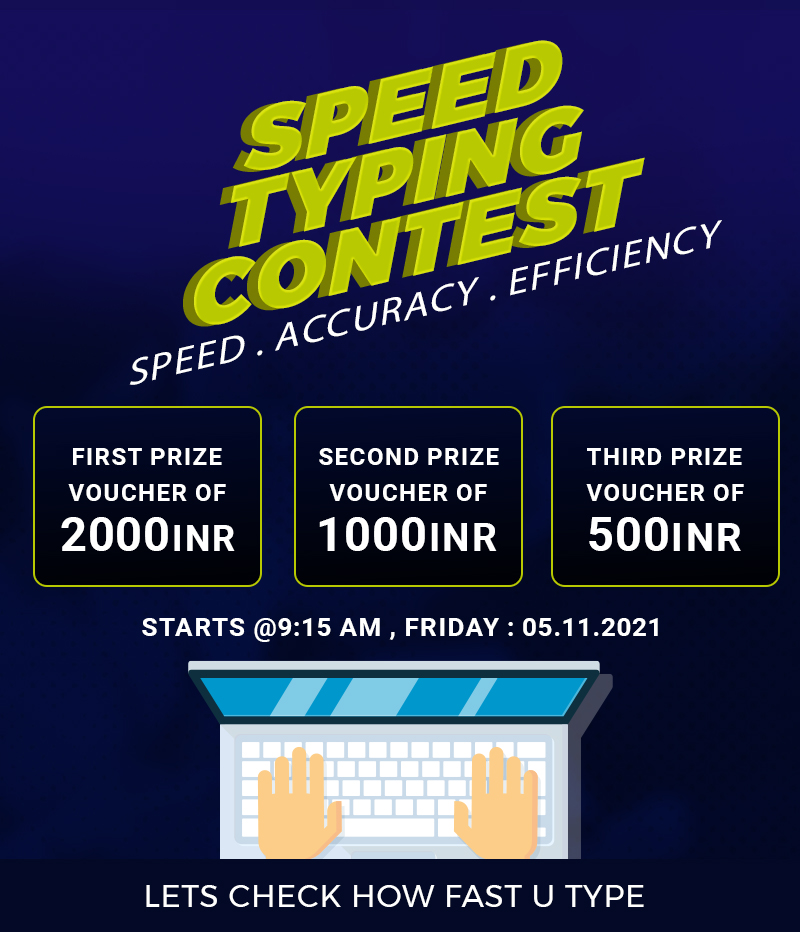The advertisement features a speed typing contest set against a dark blue background. Prominently displayed in greenish-yellow, all-capital letters are the words "SPEED TYPING CONTEST," angled toward the upper right corner. Beneath this, in all caps and white letters, is the text "SPEED. ACCURACY. EFFICIENCY.," also tilted toward the upper right. Centrally aligned are three equally-sized boxes, each bordered with a thin greenish-yellow line. The left box announces the "FIRST PRIZE VOUCHER OF 2000 INR," the middle box details the "SECOND PRIZE VOUCHER OF 1000 INR," and the rightmost box states the "THIRD PRIZE VOUCHER OF 500 INR." Below the prize details, white text indicates the contest starts at 9:15 AM on Friday, May 11th, 2021. Further down, a white keyboard connected to a laptop with a blue screen is depicted, with hands positioned on the keyboard, emphasizing the typing theme. At the bottom, in all white capital letters, the image concludes with the challenge, "LET'S CHECK HOW FAST YOU TYPE." The overall image quality is clear, with ample lighting making all elements easily visible.